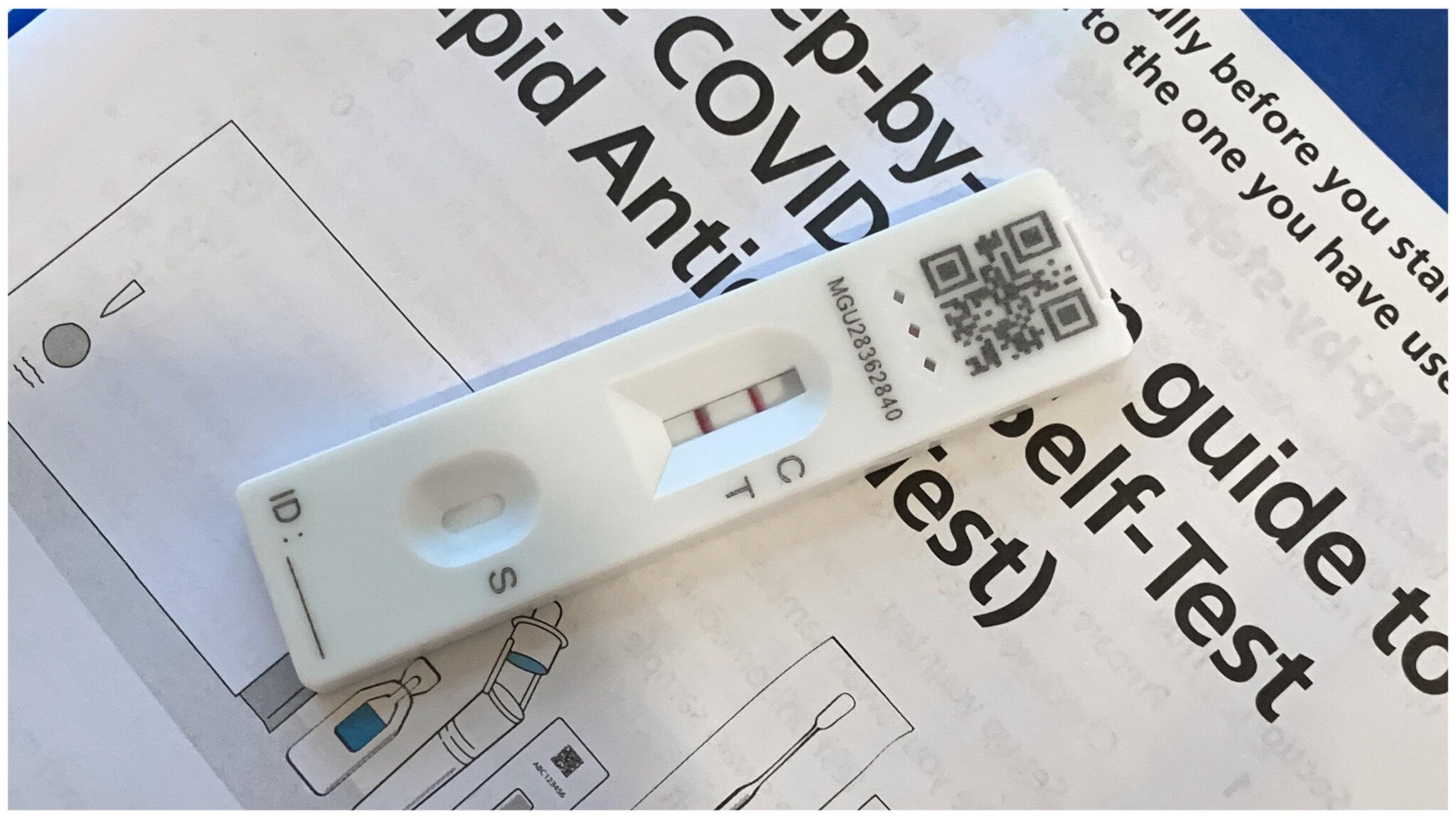This close-up image provides a detailed aerial view slightly angled from the side. The background is a gradient of blue, transitioning from a deep, almost black hue at the top to a lighter blue before merging into the white pamphlet in the foreground. The edges of the background include two noticeable blue triangles, a small one in the upper left and a larger one in the upper right, adding a sense of dimension despite a lack of texture.

The focal point of the image is a COVID-19 instructional guide for self-administering an antigen test. Although some of the text is partially cut off, the visible bold words prominently guide readers on how to perform the test. Below the text, partially visible diagrams provide further instructions. The pamphlet is positioned diagonally, offering a glimpse of the text and images on the reverse side, likely additional guidelines for the test.

Laying diagonally across the pamphlet is the COVID-19 antigen test kit itself. It features a QR barcode at the bottom and three small diamond shapes aligned horizontally. Black alphanumeric characters are displayed across the device, with two pink lines indicating the control (C) and test (T) regions, signifying a positive result. Near the bottom of the test, an "S" is marked beside a small oval where the sample was applied. The very bottom of the test device includes a blank line labeled "ID:", meant for user identification details.